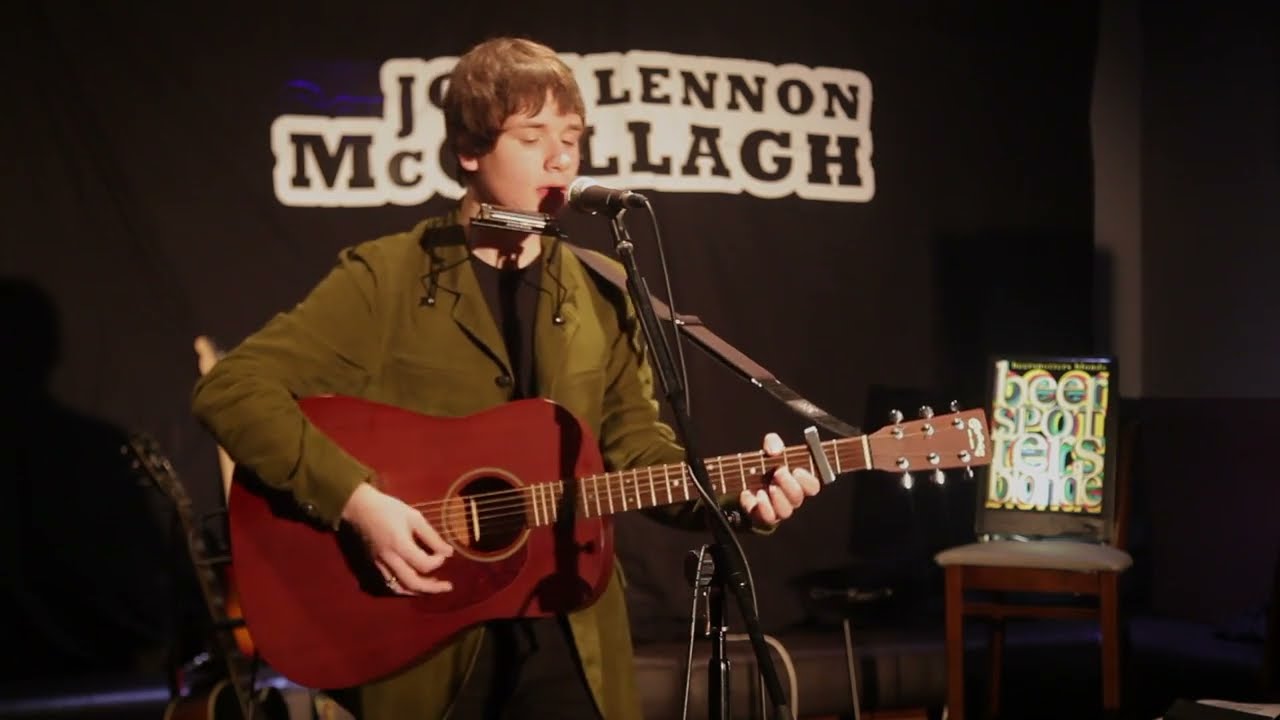The image depicts a young man, possibly in his late teens, performing on stage. He is in front of a microphone, singing with his mouth slightly open. He has light skin and shaggy brown hair, and he is playing an acoustic red guitar equipped with a capo on the neck and a strap. Around his neck is a harmonica holder with a harmonica. He is dressed in a dark, olive-green jacket with a velvet-like texture, over a black t-shirt, and matches with black slacks. Behind him, partially obscured by his head, is a backdrop that reads "John Lennon" and then "MC... L-L-A-G-H." To the left, there is a chair with what appears to be a book or poster placed on it, which has the text "beer spotters blonde" though it’s somewhat pixelated. The overall setting seems to be either a concert or a scene from a movie or TV show, with a grayish-black backdrop. There is also another guitar visible in the background.